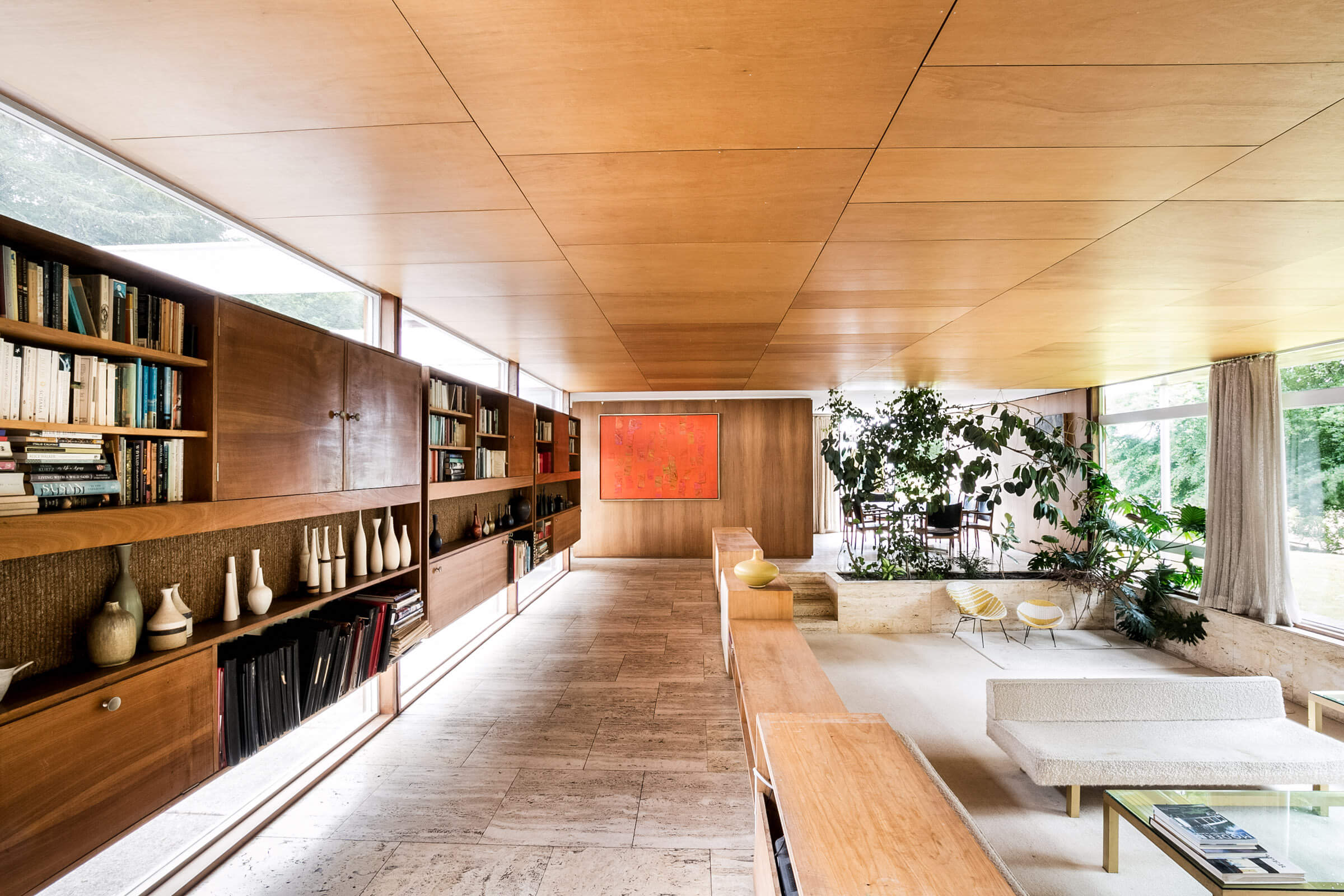This vibrant color photo showcases the interior of a modern, open-concept living space that seems to blend the functions of a living room, library, den, and dining area. The room features a light-colored, wood-paneled ceiling which enhances the brightness and adds warmth. The floor is covered in gray, polished concrete tiles that reflect the room’s modern aesthetic. 

On the left side of the room, there are several wooden shelves and cabinets, filled with a mix of books, pottery, jugs, and vases, as well as vinyl records and thin black binders, adding a touch of retro charm. The storage extends along the wall, integrating seamlessly into the overall design. 

To the right, there’s a comfortable, modern seating area consisting of white cloth chairs and a shallow, cream-colored bench positioned around a square glass table. Tall green plants line the back of the desks, reaching from the floor to the ceiling, contributing to the room’s fresh and airy feel. 

The right wall is dominated by large windows with opened drapes, allowing an abundance of natural light and offering a view of lush green vegetation and trees outside. Additionally, at the far end, there's a hint of a dining setup with a table and larger chairs, suggesting a space versatile enough for both relaxation and dining.

Finally, a red poster with various items and decorations adorns the very back wall, further accentuating the room's eclectic and personalized atmosphere.